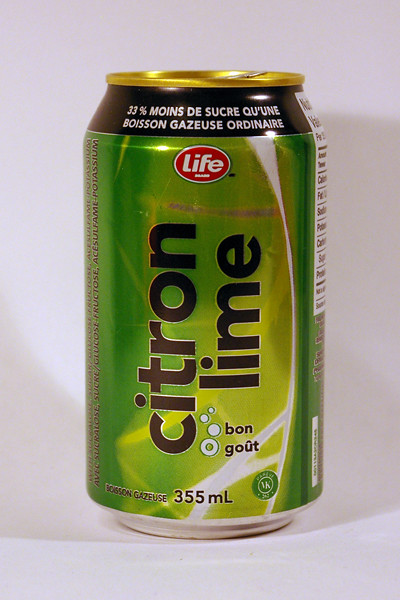The professionally photographed image showcases an aluminum soda can with a unique design. The can's top features a distinctive golden color, contrasting with the silver of the bottom. Dominantly adorned in green and yellow with a hint of white, the can sports a black top border stating "33% moins de sucre" in French, indicating reduced sugar content. Below this, within a red oval, large white letters spell out "LIFE," presumably the brand's name. 

A prominent black text "citron lime" (or "lime lemon") flavor designation appears in the can's center. The French term "boisson gazeuse ordinaire" is also present, likely describing the soda type. Scattered around the can are small circle designs that mimic bubbles, enhancing the soda theme. A nutrition label is visible at the top right, printed in black text on a white square. The text "Bong Goût" (Good Taste) with a grave accent on the "ù" adds a finishing touch to the bottom side of the can. The total volume capacity is clearly marked as 355 milliliters. The can is captured against a light background, highlighting its vibrant details.